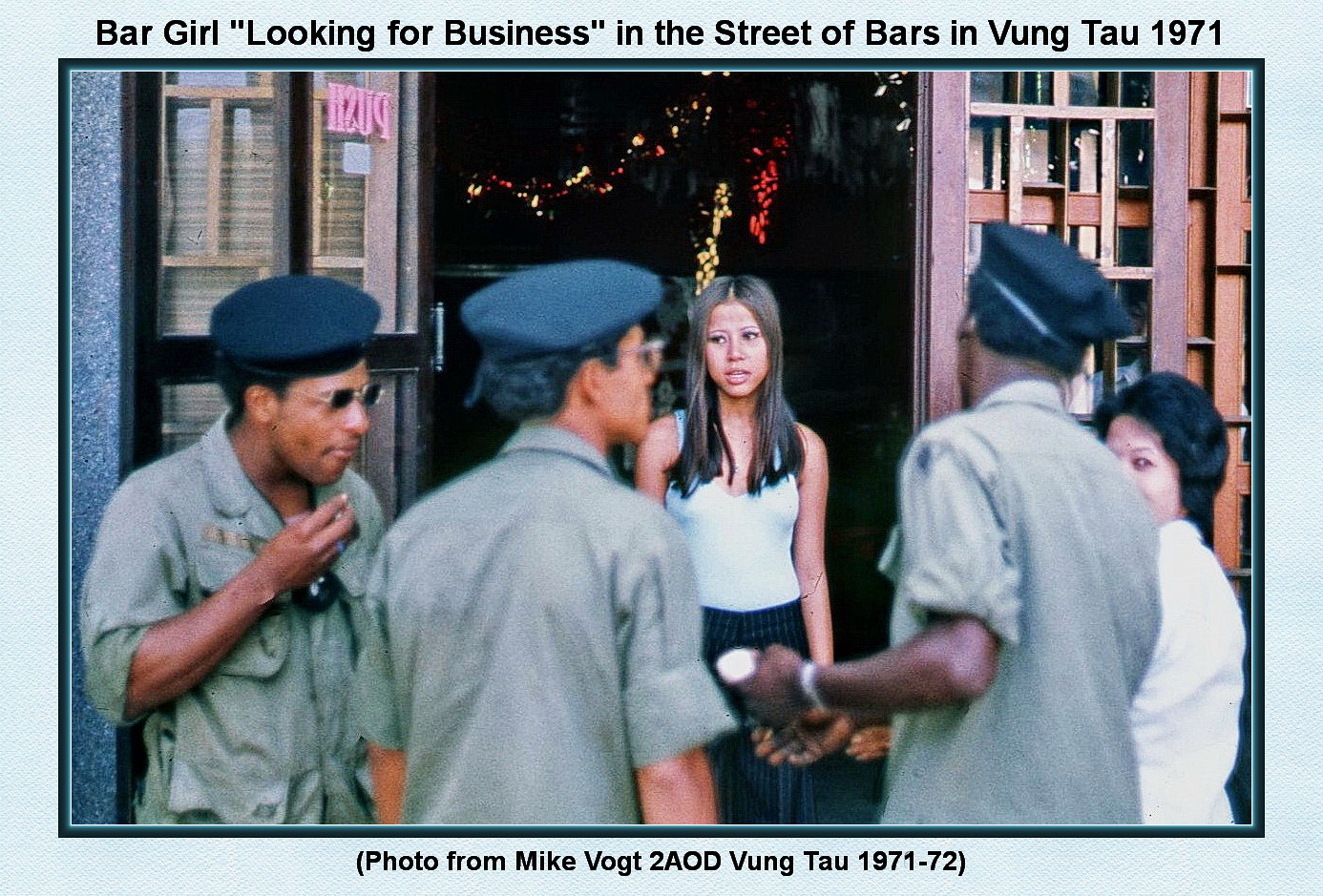The vintage image captures a scene outside a bar in the bustling "Street of Bars" in Vung Tau, 1971, during the Vietnam War. Framed by a gray border with the caption, "Bar Girl 'Looking for Business' in the Street of Bars in Vung Tau, 1971," the photo, credited to Mike Vogt, depicts a poignant moment in wartime. At the forefront, a young Asian woman with long hair, clad in a white tank top and black slacks, stands in the doorway of the bar, seemingly waiting for attention. To her side, another woman with short black hair and a white shirt interacts with soldiers donning green cargo shirts and officer caps. Among the military personnel, three African-American servicemen in berets and service uniforms, embellished with badges and name tags, are prominently visible; one, on the left, wears sunglasses. The setting appears to be a lively street, possibly lined with nightclubs or restaurants, suggested by the glowing lights within the storefront. This evocative snapshot vividly encapsulates the era, underscoring the intersection of civilian life and military presence in wartime Vietnam.